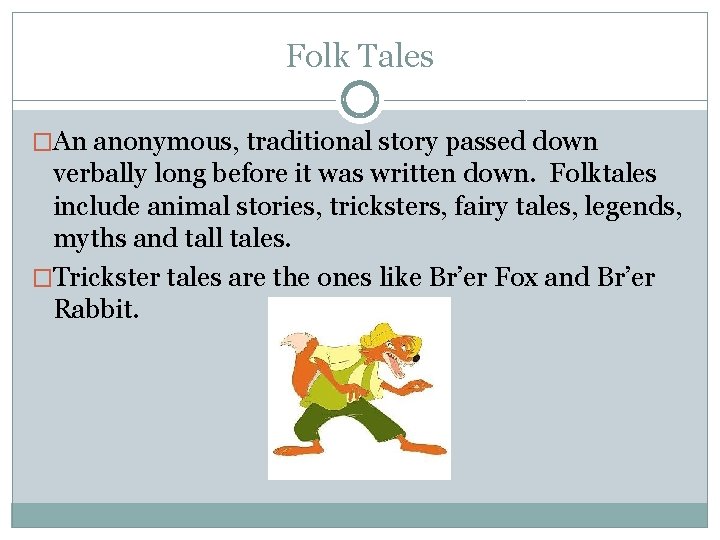The image appears to be an educational PowerPoint slide about folktales, likely intended for children. The slide's title, "Folktales," is displayed in blue letters at the top. Below the title are two red, square bullet points with black text. The first bullet point explains that folktales are anonymous traditional stories passed down verbally long before they were written down, including various genres such as animal stories, tricksters, fairy tales, legends, myths, and tall tales. The second bullet point elaborates that trickster tales, such as those of Brer Fox and Brer Rabbit, are a category of folktales.

Beneath the text, there is a white square containing a cartoonish illustration of Brer Fox. The animated depiction shows Brer Fox with an orange face, arms, and tail (the tip of the tail being cream-colored). He is dressed in a yellow straw hat, dark green pants, and a light green shirt over a white shirt. The fox is hunched over with his mouth open, showing his teeth, and his arms extended. The background colors of the slide include shades of white, blue, black, orange, and green, all well-aligned and centered, giving a polished presentation feel.